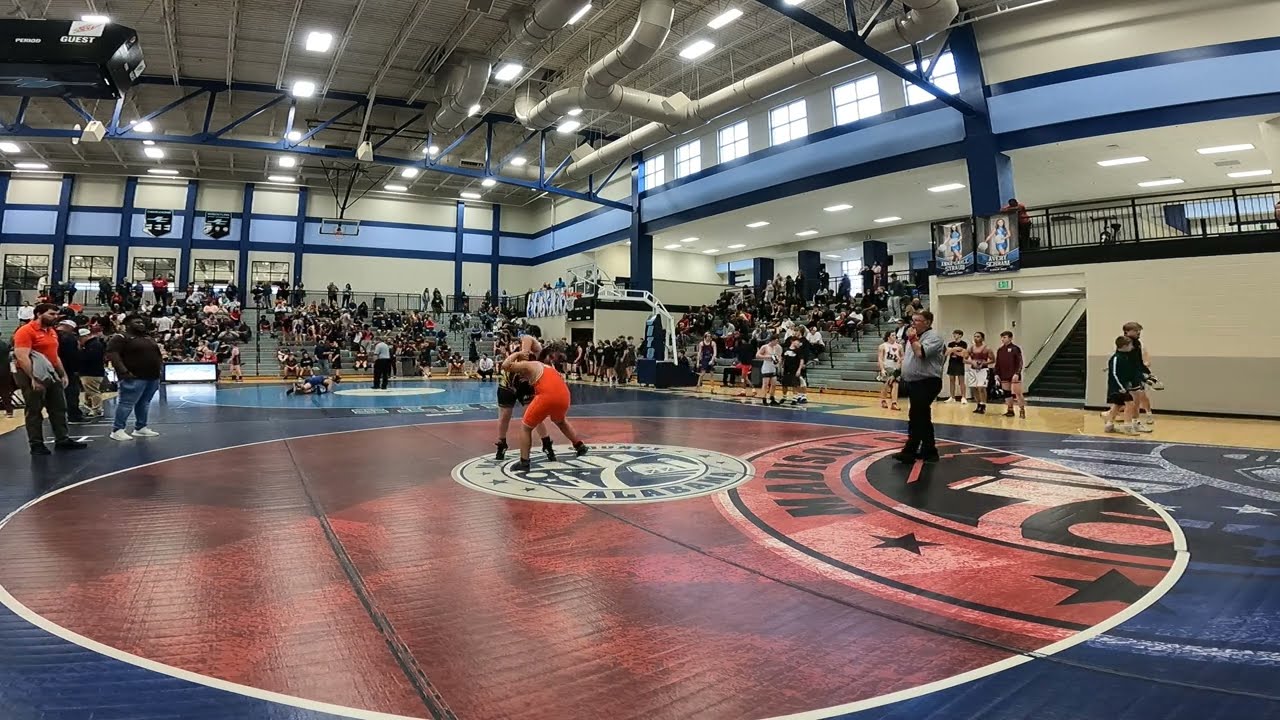The photo captures a lively wrestling meet taking place inside a school gymnasium. The gym is well-lit by numerous rectangular fluorescent lights embedded in a white ceiling, complemented by dark blue support beams. The white walls feature a blue stripe along the top, with a strip of gray at the bottom. A series of square windows on the right side allows natural light to filter into the space. In the center foreground, a small circular wrestling area is marked "Alabama" on a red background, encircled by blue. Two wrestlers, one in black and the other in an orange sleeveless leotard, are intensely grappling. The wrestler in orange is bent over, fully engaged in the match. Nearby, a referee in black pants and a gray short-sleeved shirt closely monitors the bout, holding a whistle to his mouth. Surrounding the main action, the bleachers are nearly two-thirds full, bustling with spectators and teeming with energy. Coaches and team members, some wearing distinctive orange and black outfits, stand anxiously on the sidelines, deeply invested in the competition. In the background, another wrestling match is also in progress, featuring two grapplers on the floor, indicating multiple matches happening simultaneously in this bustling gym.